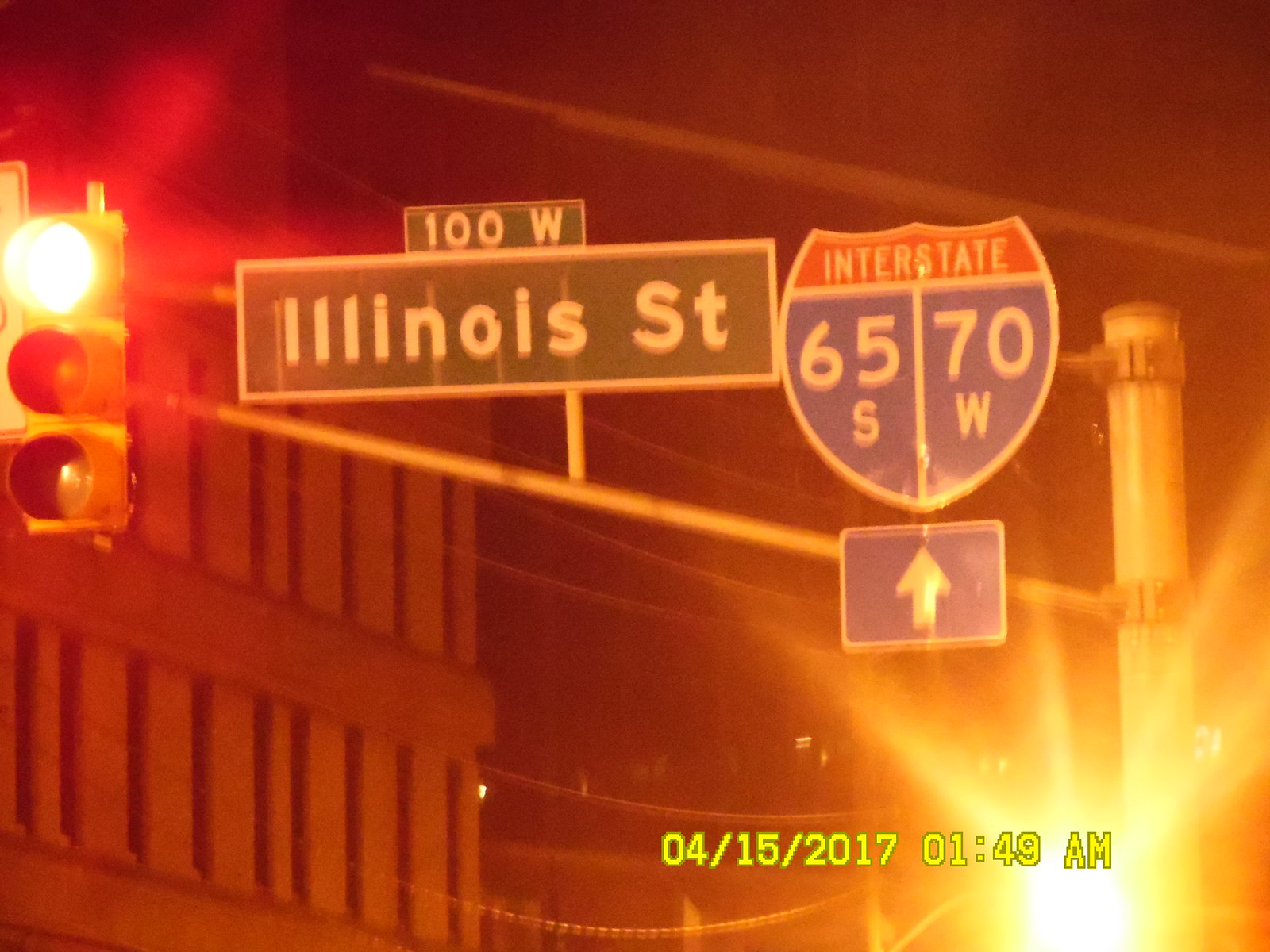This nighttime photograph, slightly out-of-focus and low in quality, captures a traffic scene dominated by various street and interstate signs mounted on a horizontal pole, connected to a large vertical pole on the right side. Prominently displayed is a green street sign reading "Illinois Street," with a smaller green sign above it indicating "100 West." To the right of these signs is a shield-shaped interstate sign showing "65 South" and "70 West," accompanied by a blue sign with an upward arrow beneath it. The upper left corner features a traffic light, glowing red. In the background, a street light causes noticeable lens flares that blur parts of the image. Additionally, a timestamp is visible in the lower right corner, displaying "04-15-2017 01:49 AM." The ambient lighting from the street and surrounding buildings adds to the scene's nocturnal ambiance.